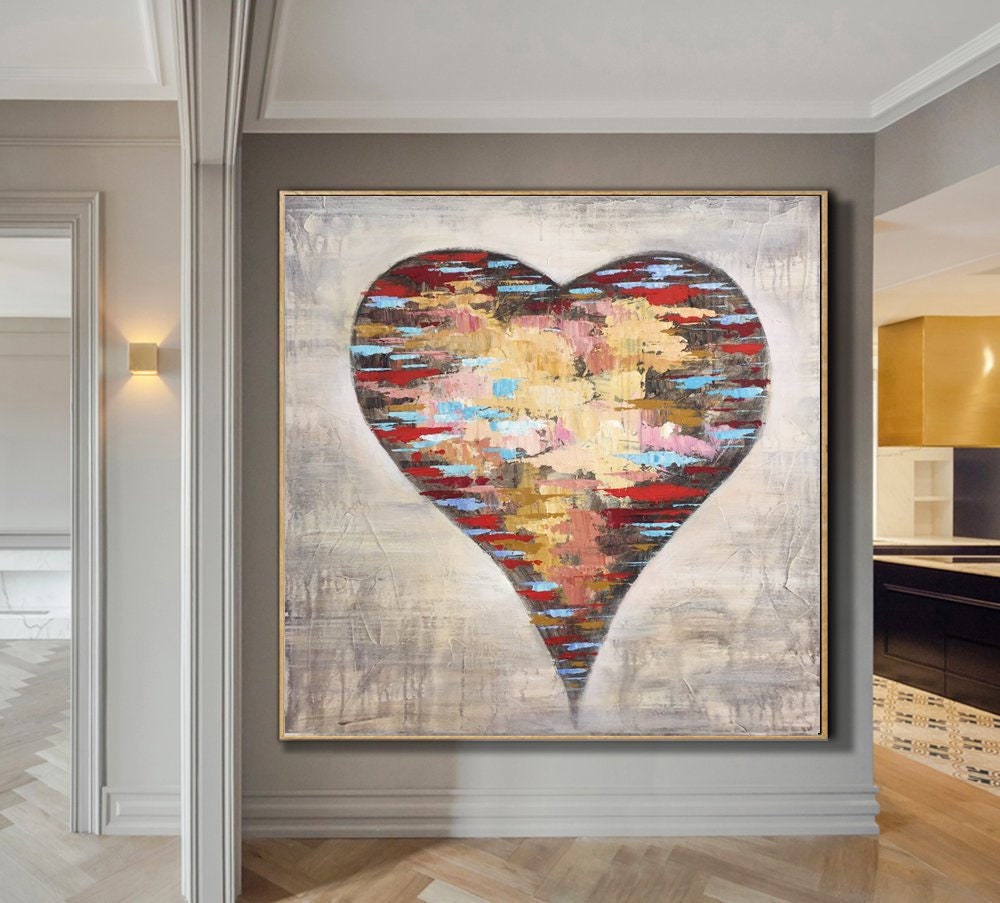The image depicts a large, framed artwork hung on a gray wall within a domestic interior, possibly a house or apartment. The room features wood flooring and a section of tile floor to the right, suggesting a nearby kitchen. A small light fixture is mounted on the wall, illuminating the scene, with glimpses into an adjoining room to the left.

The focal point of the image is an eye-catching, massive painting almost spanning the height of one wall. This painting, set in an ornate gold metal frame, portrays a heart at its center. The heart is composed of smeared and overlapping hues of red, blue, pink, yellow, gold, light blue, and tan, creating a vibrant and chaotic palette. The heart tapers to a distinct point at its base.

The background of the painting, a blend of gray and white tones, appears drippy and somewhat amorphous, evoking blurred images that resemble a cityscape or an abstract conglomeration of houses and trees. The overall aesthetic of the artwork is one of spontaneous, layered brush strokes, imparting an impressionistic and somewhat amateurish feel.